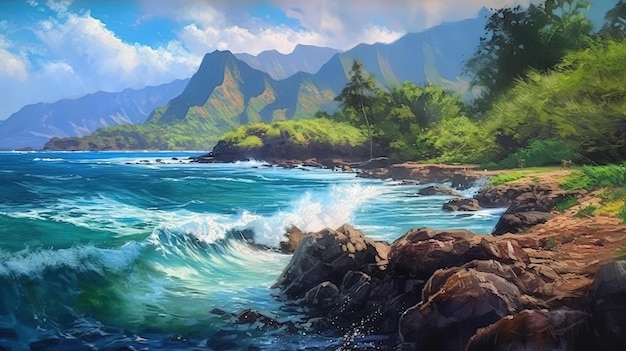The painting depicts a serene yet dynamic coastal landscape, capturing the interplay of nature's elements in vivid detail. On the left side, vibrant choppy waves in varying shades of deep blue and green crash energetically onto the rock-strewn shore, their white caps turning into bubbly foam upon impact. The rocky shoreline extends to the center and right side, characterized by realistic brown rocks interspersed with patches of green grass and weeds. Above this rugged terrain, light and dark green foliage adds texture to the scene.

Dominating the upper section of the painting is a strikingly realistic light blue sky, filled with puffy, drifting clouds, enhancing the sense of depth and tranquility. In the far distance, a majestic mountain range stretches across the horizon from left to right, with colors transitioning from blue-gray to dark gray and even hints of green and orange, enriching the visual palette.

The entire scene is bathed in natural light, devoid of any human presence or text, presenting a pure, unspoiled outdoor vista where water, land, and sky converge harmoniously.